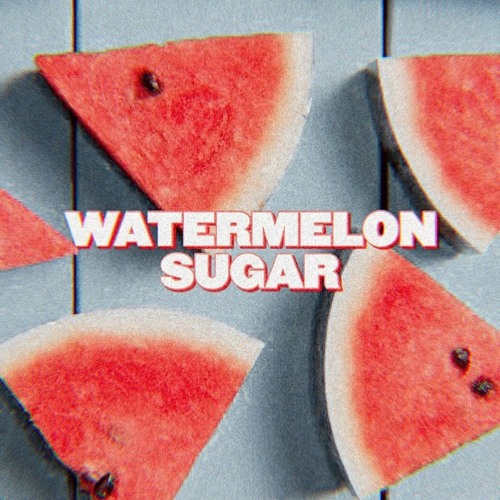The image displays what appears to be an album cover for "Watermelon Sugar." The background features gray, slatted deck boards or possibly a picnic table crafted from a composite material. Arranged on these deck boards are five watermelon slices, cut into triangular shapes, revealing rich dark pink flesh contrasted by white rinds. Each slice contains a few black seeds, noticeable but not overly abundant, which gives them the characteristic appearance of seedless watermelon. 

The slices are strategically positioned, with some being partially cut off by the image border, while others are fully visible. Across the middle of the image, the title "Watermelon Sugar" is prominently displayed in bold white letters accented with pink shadows, adding depth to the text and ensuring that it stands out against the background. The overall composition and detailing of the image suggest that it is designed with artistic intent, likely to serve as an eye-catching and thematic album cover.